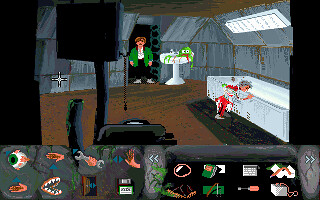The image depicts a cartoon-style video game screen from a computer. Central to the scene is a man dressed in a green jacket, white shirt, black pants, and white shoes, stepping out of a doorway and moving towards the camera. To his right, there's a white sink with a small, green creature lying motionless inside. Further right, a long, white table stretches vertically along the image, over which a person appears to be bending down, surrounded by a significant amount of red, suggesting they might be deceased. At the bottom of the screen, a menu bar displays various icons including an eyeball, a mouth, a hand, a pair of pliers, a disc, a door, another hand, and several items on a black background that are hard to discern but might include a credit card, a silver box, and a screwdriver. Additionally, a black computer screen is positioned to the right, facing away from the viewer toward the man coming through the door.